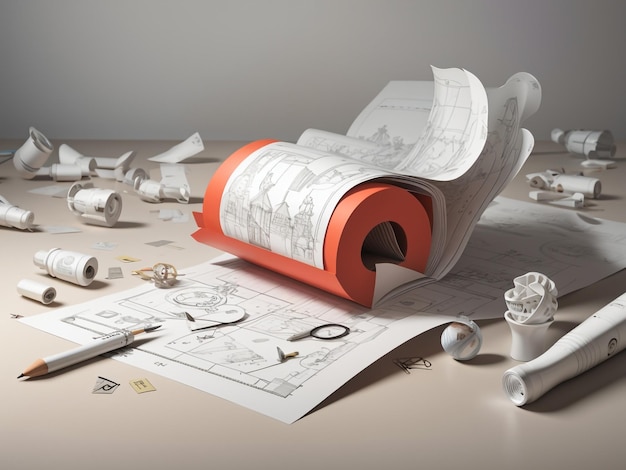The image reveals a possibly AI-generated or photorealistic surreal depiction of an architect's desk. The desk, a white table with a semi-matte surface, is strewn with various supplies and unusual objects. Central to the scene is a terracotta-colored cylindrical dispenser, from which architectural sketches unfurl, displaying detailed pencil drawings of buildings and cities. Scattered around are white objects, including a peculiar white pencil that resembles a toothpick at one end, a small sake glass with a twisted, smashed ping-pong ball inside, and something akin to the handle of an aluminum baseball bat, but in white. Also present are a beige light-gray surface beneath the items, several cylindrical shapes, black paper clips, and small tags. The background is a monochrome gray or white wall. The surreal arrangement of objects, most of which appear randomly placed and difficult to identify, contributes to an overall sense of disarray and abstraction, suggesting a complex, labor-intensive workspace.